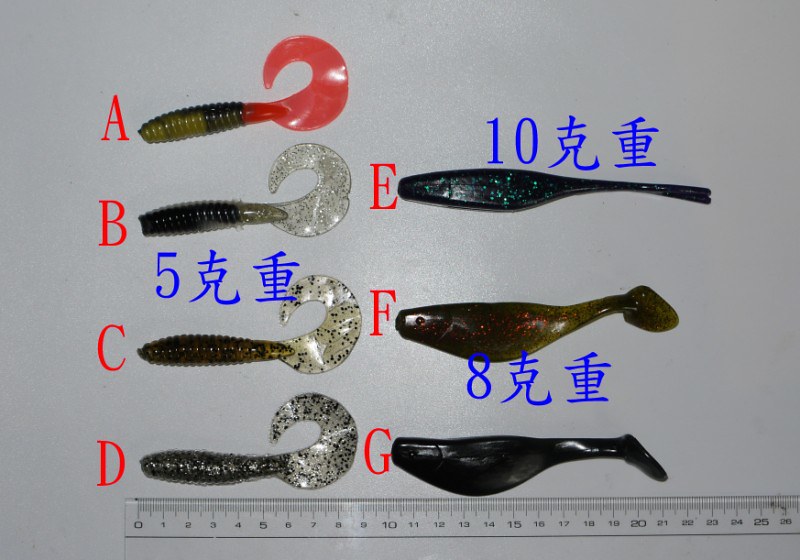This indoor color photograph showcases a meticulously arranged collection of seven fishing lures displayed on a white countertop. The lures are organized in two columns; the left column features four lures labeled A, B, C, and D, while the right column has three lures labeled E, F, and G, all marked with red letters. These lures vary in shape, with three distinct types: some feature a curly-Q tail, others have long, thin tails, and a third type has thicker tails. The lures come in glittery shades of blue, brown, black, and white, with one curly-Q tail lure sporting a striking red tail. Additionally, some lures resemble small fish or guppies. Below this orderly display, a clear ruler marked in millimeters indicates their size. Scattered along the display are numbers and Chinese characters, possibly denoting prices, with blue numbers 5, 10, and 8 positioned near the characters.